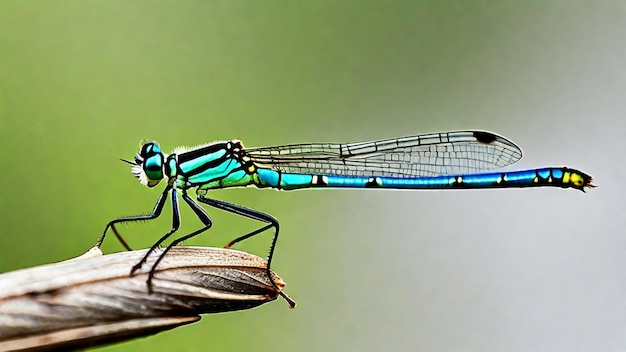The image shows a vibrant dragonfly, primarily colored in shades of blue, turquoise, green, and yellow, facing towards the left. Its elongated body features distinct segments: the end of the abdomen is yellow, transitioning to blue and turquoise sections separated by black and white lines. The head is teal with large, striking green and black eyes, covered in light hair, giving it a fuzzy appearance. The dragonfly's delicate, translucent wings, adorned with geometric patterns and small black lines, are positioned along its abdomen. It perches on an oval-shaped, tan and black leaf that enters the image from the bottom left and becomes more focused near the dragonfly's body. This dragonfly's six thin black legs grasp the leaf firmly. The background is a soft blur of green and white hues, with a more saturated green in the upper left and whitish-gray tones in the lower right, emphasizing the dragonfly's detailed, colorful form.